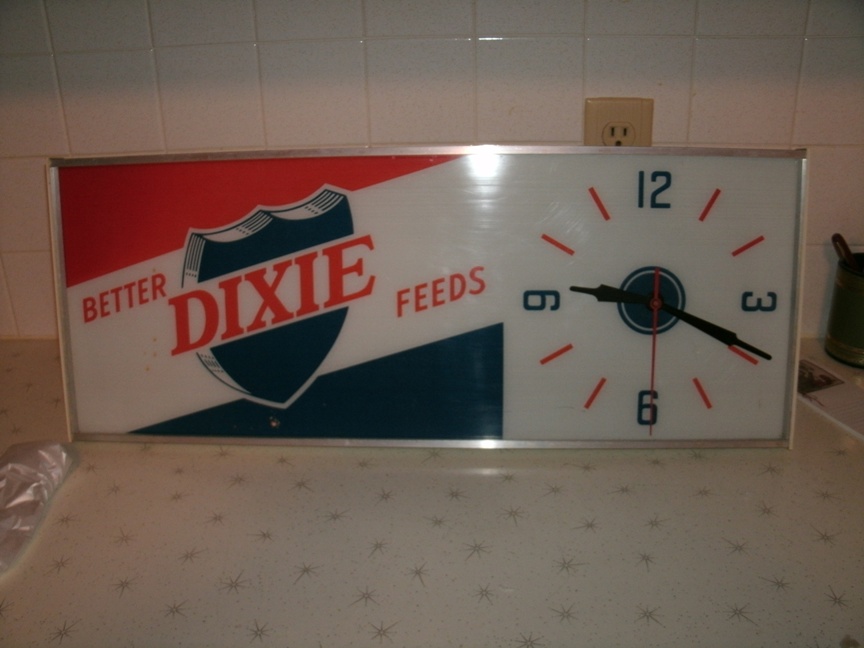This photograph captures a vintage advertising backlit analog clock, likely from the 1970s to the 1990s, sitting on a beige countertop speckled with dark grey starburst patterns. The clock, trimmed in a silver aluminum frame, leans against a white tiled wall that includes a small beige electrical outlet. The rectangular clock features a prominent logo on the left side, displaying "Better Feeds Dixie" in red text over a blue shield with a diagonal white stripe, dividing blue and red corners.

The clock face on the right side is predominantly white, showcasing dark blue numbers at the 12, 3, 6, and 9 positions, while red lines mark the other hours. In the center, there are blue clock hands for the hour and minute, alongside a contrasting red second hand. The backlit nature of the clock enhances its visibility, reflecting its translucent front which further emphasizes its vintage appeal. Off to the left of the clock on the countertop, a small piece of foil is visible, and an indistinct object sits to the right, adding contextual detail to the setting.